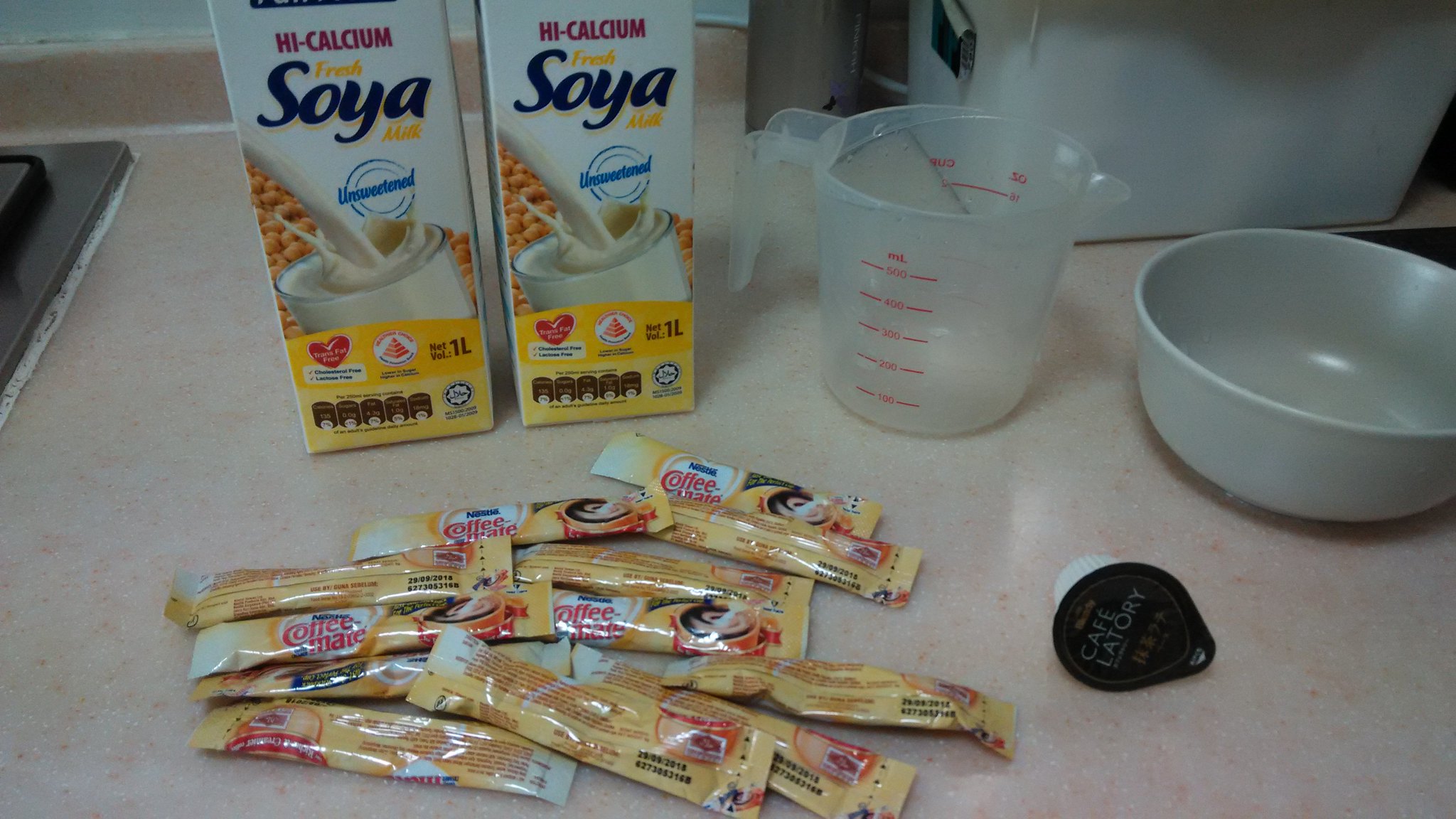This photograph, taken from above, captures a detailed view of a kitchen countertop with a light white and pinkish surface. Prominently situated are two identical 1-liter cartons of high calcium, unsweetened fresh soy milk, each decorated with an image of milk pouring into a glass, creating a rippling effect. In the upper background, a white box is visible. To the right of the cartons is a clear plastic measuring cup with a pourable handle, alongside a small white bowl. Scattered across the counter are numerous yellow individual serving packets of Coffee Mate creamer. To the left of these items is a single K-cup with a black top, labeled Cafe Latorre. Peeking from the upper left edge of the image is a stainless steel stove, adding context to the kitchen setting.